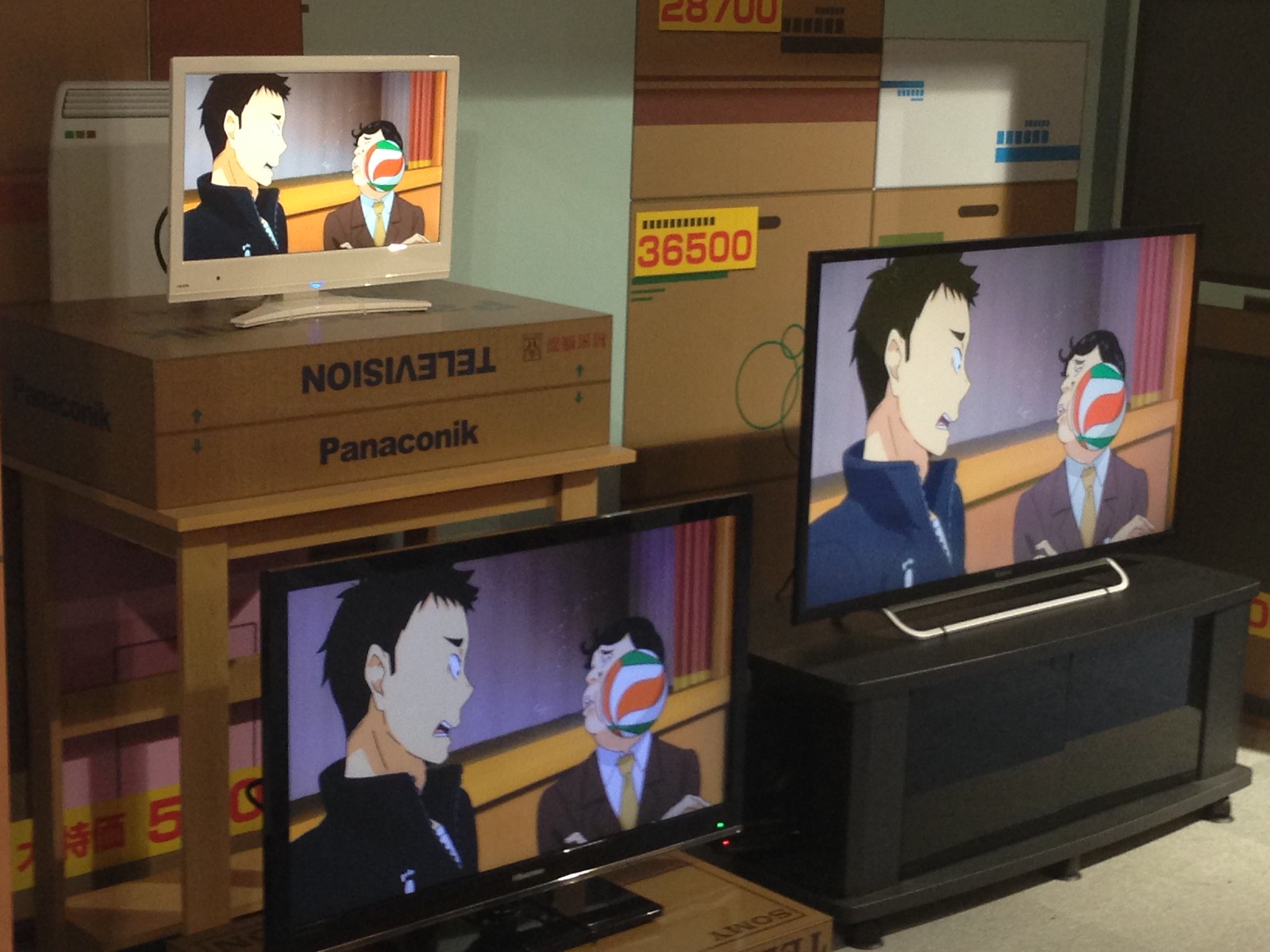This photograph depicts a television store, showcasing three different flat screen televisions of various sizes. The TVs are displayed on stands and boxes, each illustrating the same anime scene. To the left, the smallest TV resembles a computer monitor with a white trim, resting on a brown box labeled "television" upside-down, and "PANACONIK" (a misspelling of Panasonic). The middle TV, larger and framed in black, also sits on a box. The largest TV is positioned to the right on an entertainment stand, with brown boxes and yellow price signs showing figures such as 36500 and 28700 surrounding it.

The anime scene is the same on all three screens: two men are in focus. The man on the left, who has black hair, triangular brows, a small nose, pale skin, and a black zip-up jacket over a white shirt, displays an expression of surprise. His mouth is open and drawn downward as if recoiling. The second man, standing to the right, is being hit in the face by a volleyball with red, white, and green colors. He has black hair, closed eyes, and is wearing a gray suit with a yellow tie. This man’s head is reeling back from the impact.

Overall, the scene in the store conveys an organized display of televisions for sale, each broadcasting a dynamic anime moment in unison.